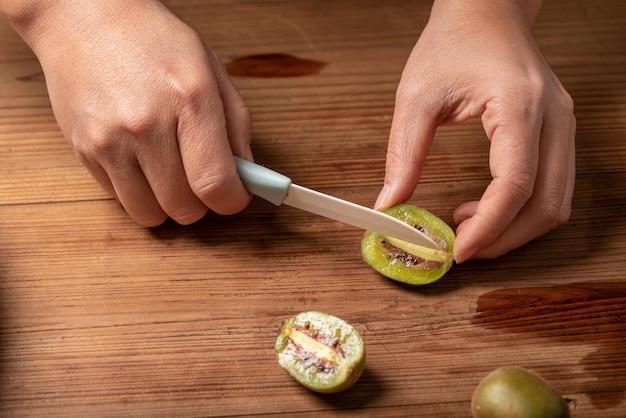The image showcases a close-up of an adult, likely a white person, cutting a kiwi fruit on a wooden surface. The scene captures both of the person's hands: the right hand holds a small knife with a light blue handle and a white blade, poised to slice further into a halved kiwi held by the left hand. The kiwi is small, almost the width of the person's index finger and thumb. The cutting action appears to be taking place on a wooden board or table. In the foreground, apart from the kiwi being cut, there are two additional kiwis: one halved and showing its typical bright green interior, and another whole with its characteristic brown, hairy skin. There are also subtle water stains visible on the wood, adding to the realistic nature of the scene.